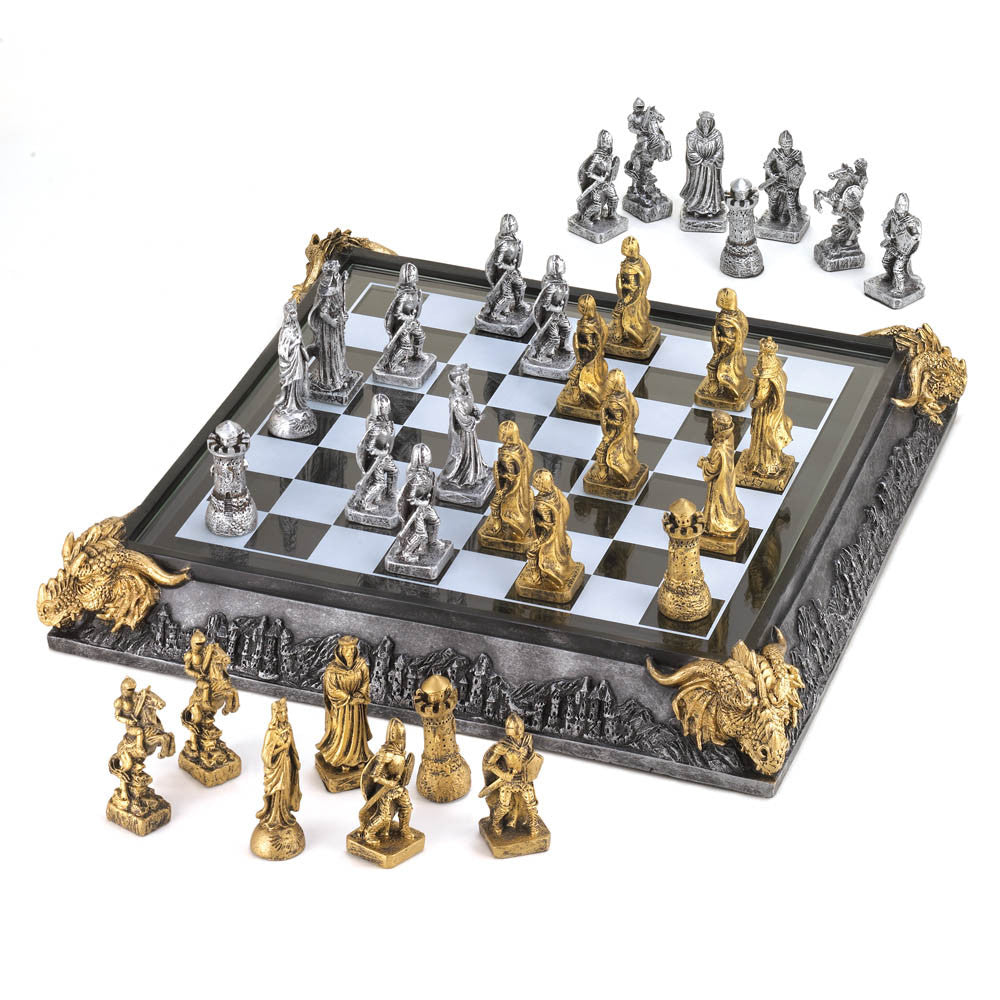The image features an intricately designed fantasy-themed chess set with gold and silver pieces. Positioned on a checkerboard with alternating light blue and dark blue (or black) squares, the board is slightly angled in the picture, suggesting an ongoing game. The gold pieces occupy the right side, while the silver pieces are on the left. The chessboard is elevated on a platform with an elaborate border that includes gold-horned dragon heads at each corner. Detailed engravings and carvings on the gray metal base give the set a medieval, Lord of the Rings-esque aesthetic. The chess pieces themselves resemble actual figures, including knights, human beings in robes and uniforms, and towers, all appearing to be crafted from painted pewter, adding a polished metallic look to the entire setup. The background of the image is plain white, further emphasizing the ornate and fantastical nature of the chess set.